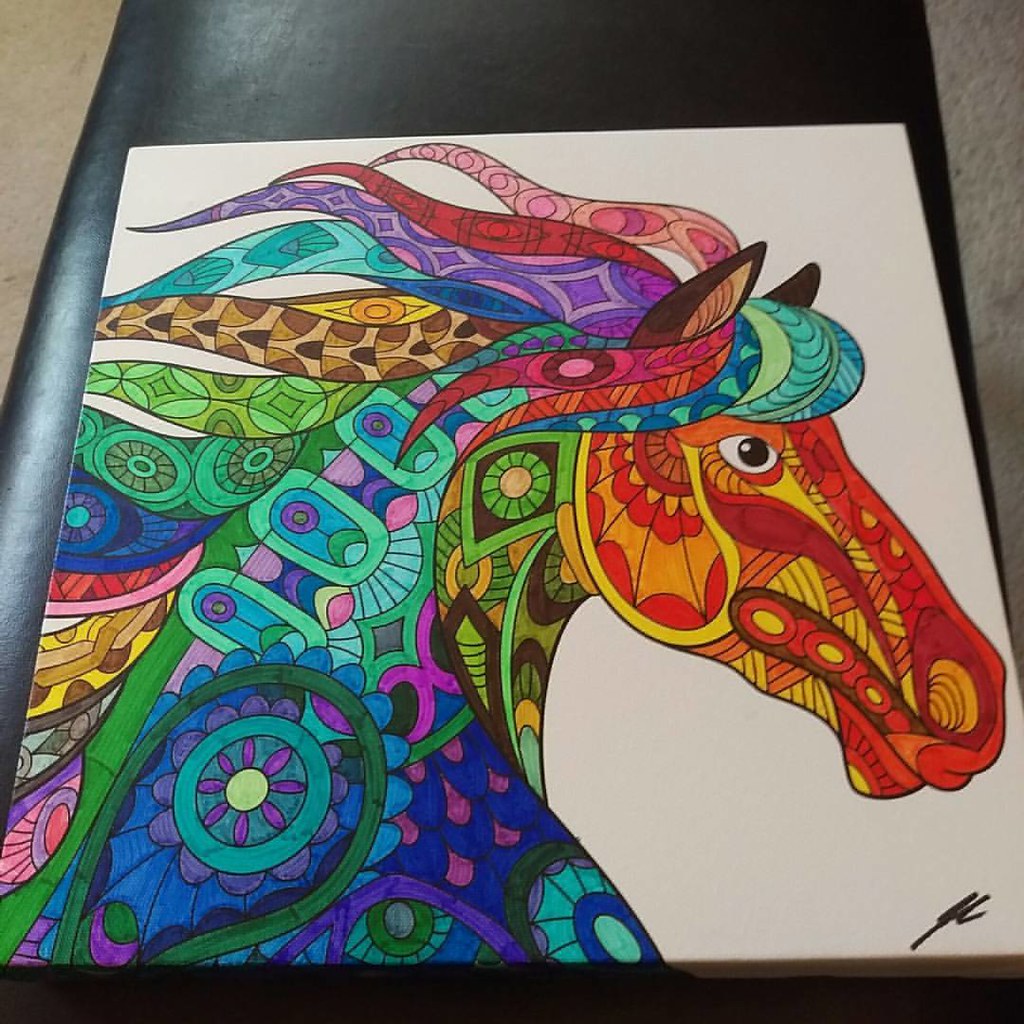This vibrant artwork depicts a stylized horse rendered on a square canvas, showcasing a meticulous blend of colorful markers. The horse's outline is crisply drawn, highlighting its striking mane. The artist employs an array of vivid colors, including red, orange, yellow, green, blue, purple, and brown, across the entire image. The horse's face, especially around the eyes and mouth, is dominated by warm hues of red, orange, and yellow. In contrast, the body is enveloped in cooler shades of blues and purples. The mane is a dazzling tapestry of mixed colors and geometric shapes, such as flowers and diamonds, creating a visually rich and dynamic composition.